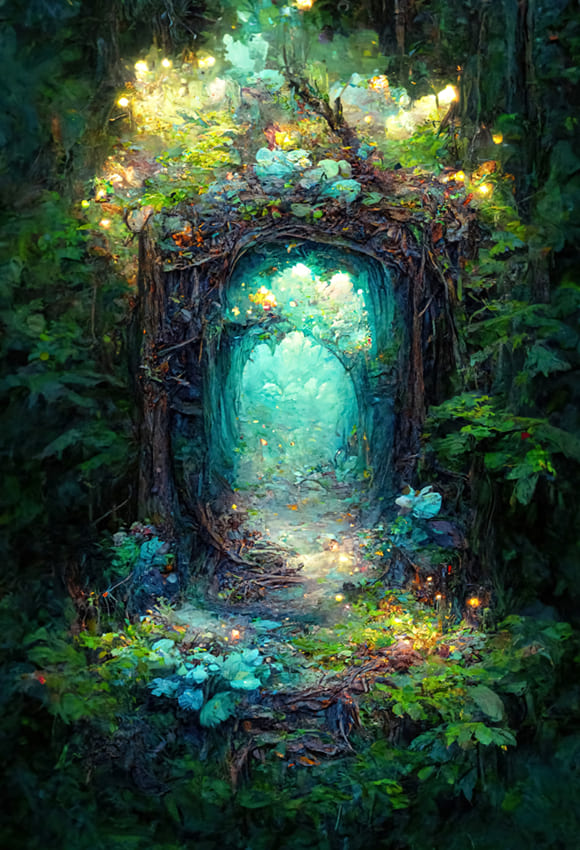The image depicts a detailed painting of an enchanted forest, featuring a tunnel-like gateway formed by vine and tree branches intertwining to create a rounded arch. This gateway is surrounded by a dense and thick forest abundant with various plants, including green ferns, blue and yellow plants, and other vibrant flora. The scene exudes an ethereal quality with an unusual light source that doesn't appear natural, radiating within and around the entrance of this natural tunnel. At the top of the arch, some flowers and plants glow with an almost magical luminescence, casting a light greenish hue inside the tunnel. The background behind this illuminated gateway remains shrouded in darkness, enhancing the mysterious and enchanted atmosphere of the forest. The entire image is crafted in a rectangular shape, blending characteristics of both a painting and a processed photograph.